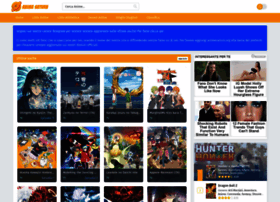A small, visually intricate website is depicted. The very top of the page is quite blurred, making the text unreadable. In the upper left corner, there is an orange sign accompanied by an orange symbol. Adjacent to this is a search bar, and further to the right, in the upper right corner, there is an orange circle with a gray circle next to it. Below these elements is an orange strip, which in turn is followed by a darker blue box displaying some white text. Beneath this blue box lies another orange box containing a clickable white box.

The main content area hosts a series of illustrated images featuring a variety of subjects in diverse colors. One image is predominantly orange and depicts cartoon characters. Another shows a person with a white face and black hair, surrounded by characters in green and yellow attire. There's also an image featuring a brown circle against a blue sky.

On the right side of the page, there is a column of smaller images, primarily portraits of people, each paired with black and white descriptions underneath. Among these is a gray-based box labeled "Hunter."

The website's design is vibrant and characterized by a combination of playful illustrations and structured content areas, yielding a colorful and engaging interface.